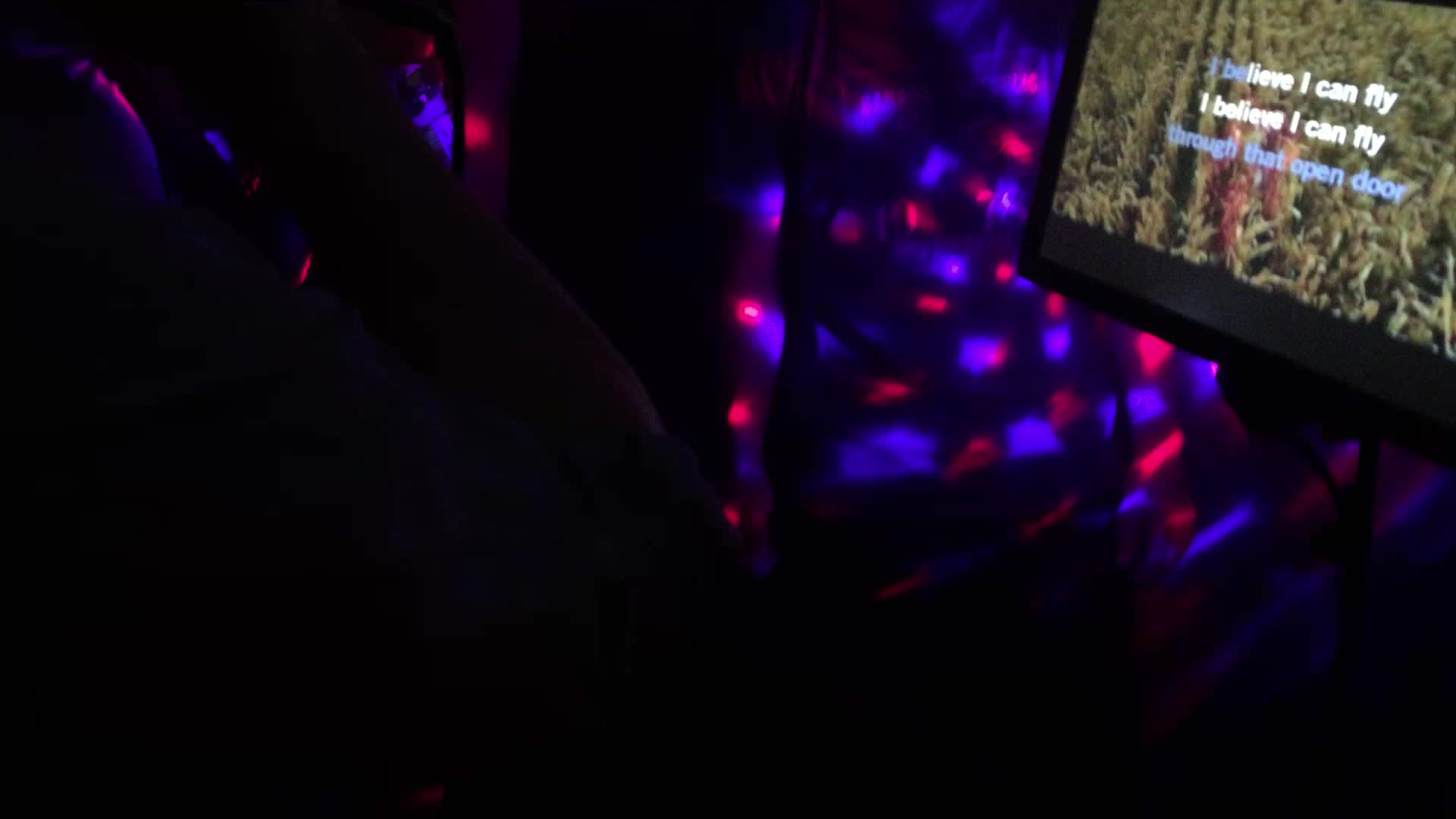This color photograph, taken inside a dimly lit bar or karaoke club, is predominantly engulfed in darkness. The only light in the scene comes from red, blue, and purplish-pink projections casting hues onto the back wall. On the upper right-hand side of the image, a monitor stands out with karaoke lyrics displayed on its screen: "I believe I can fly. I believe I can fly through that open door." The rest of the room is barely discernible, with only faint shadows hinting at the presence of other objects or people. In the far upper left-hand corner, there might be a person’s arm, adding a subtle human element to the otherwise obscure surroundings.